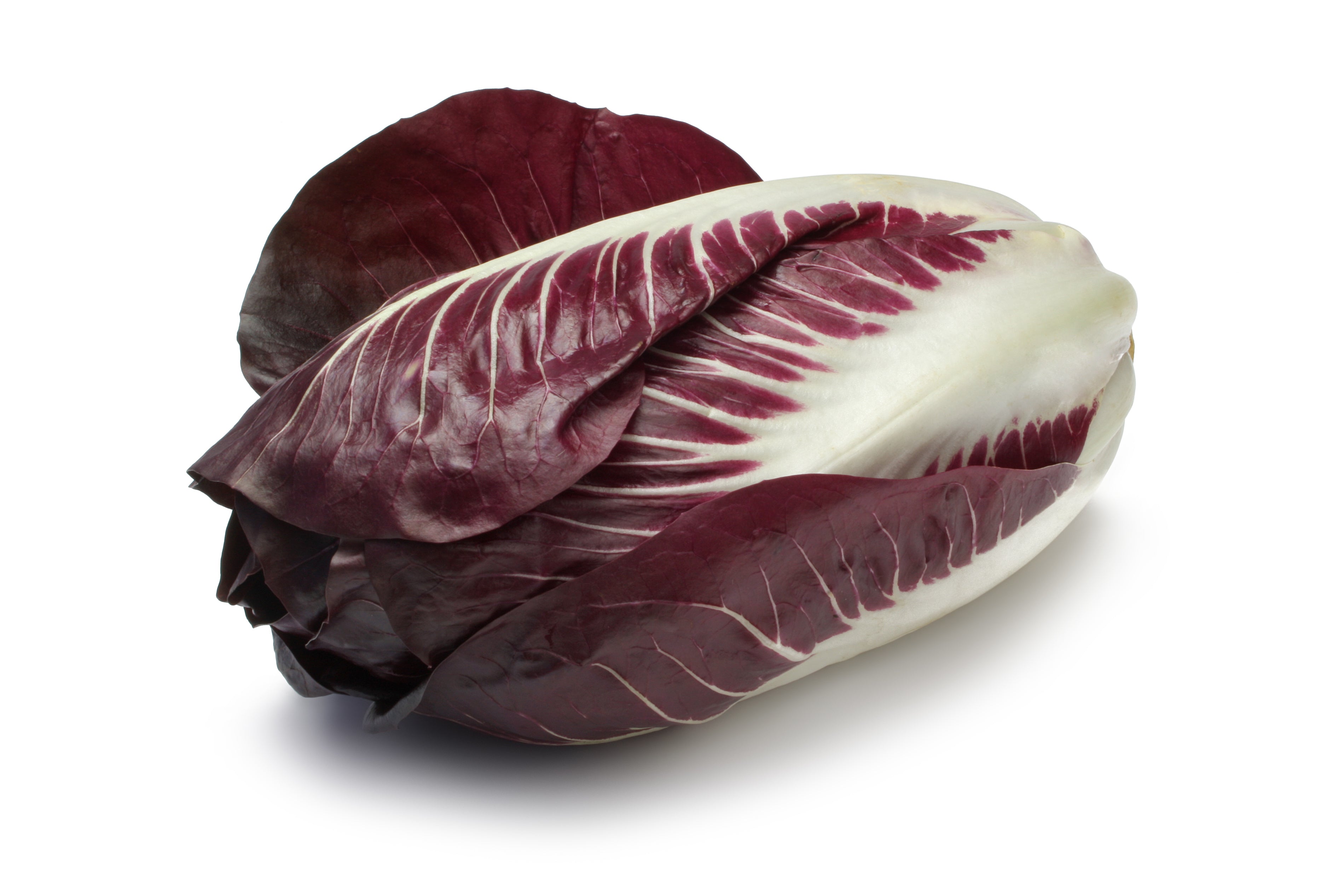A detailed photograph captures a red cabbage, exhibiting a deep purplish-red color with prominent white veins branching throughout the leaves. Resting obliquely on a pristine white surface, the shadow cast beneath it suggests light coming from above and behind. The cabbage is not perfectly round but rather oblong, with the stem end pointing towards the upper right and the leafy end extending towards the lower left. The intricate pattern of the leaf veins stand out vividly against the darker background of the leaves, giving the cabbage a striking visual complexity. Notably, one leaf protrudes prominently from the back, displaying its veining in a paler hue.